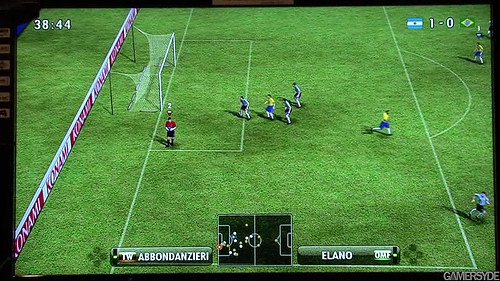The image is a screen capture of a live soccer game, displaying a pivotal moment on the pitch. In the upper left corner, the game clock reads 38:44. The upper right shows the scoreline: Argentina leading Brazil 1-0. The expansive green field features a clearly marked white rectangular penalty box near the left-side goalpost. Inside the penalty area stands a referee in a red jersey and black shorts. Near the goalpost, four soccer players are sprinting towards the goal, while another player in a yellow jersey and blue shorts can be seen running towards the right side of the field. Along the bottom of the screen, the name "ABBONDANZIERI" appears on the left, likely indicating the Argentine goalkeeper, and "ELANO" on the right, who is presumably a Brazilian player. The lower right corner of the screen shows the text "GAMERSIDE," suggesting either a broadcast watermark or video game branding.